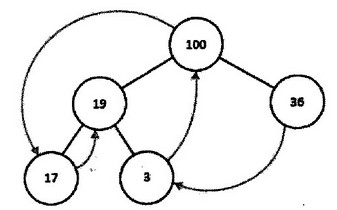This is a detailed computerized diagram featuring a set of numbered circles interconnected by directed arrows, forming a structured, triangular pattern. At the base of the triangle, there are two circles: the left circle contains the number 17, and the right circle contains the number 3. These two circles are connected by lines that direct attention towards the apex of the triangle, which holds the number 19.

From the top circle (19), lines extend outward and connect to two additional circles situated further out from the triangle's base. The left of these external circles contains the number 100, while the right contains the number 36. The arrows illustrating the directional flow within the diagram map a clear interaction between these elements.

Specifically, an arrow from the circle containing 100 points downward towards the circle with 17. From the 17 circle, an arrow then rises upward to the 19 circle. Concurrently, the 3 circle at the lower right base has an arrow extending upwards to the 100 circle. Finally, from the 36 circle, an arrow directs downward towards the 3 circle, encapsulating the cyclical or interdependent nature of the relationships depicted.

Each connection signifies a directional influence or interaction between the numerals, providing insight into the dynamic processes or relationships that the diagram is intended to represent.